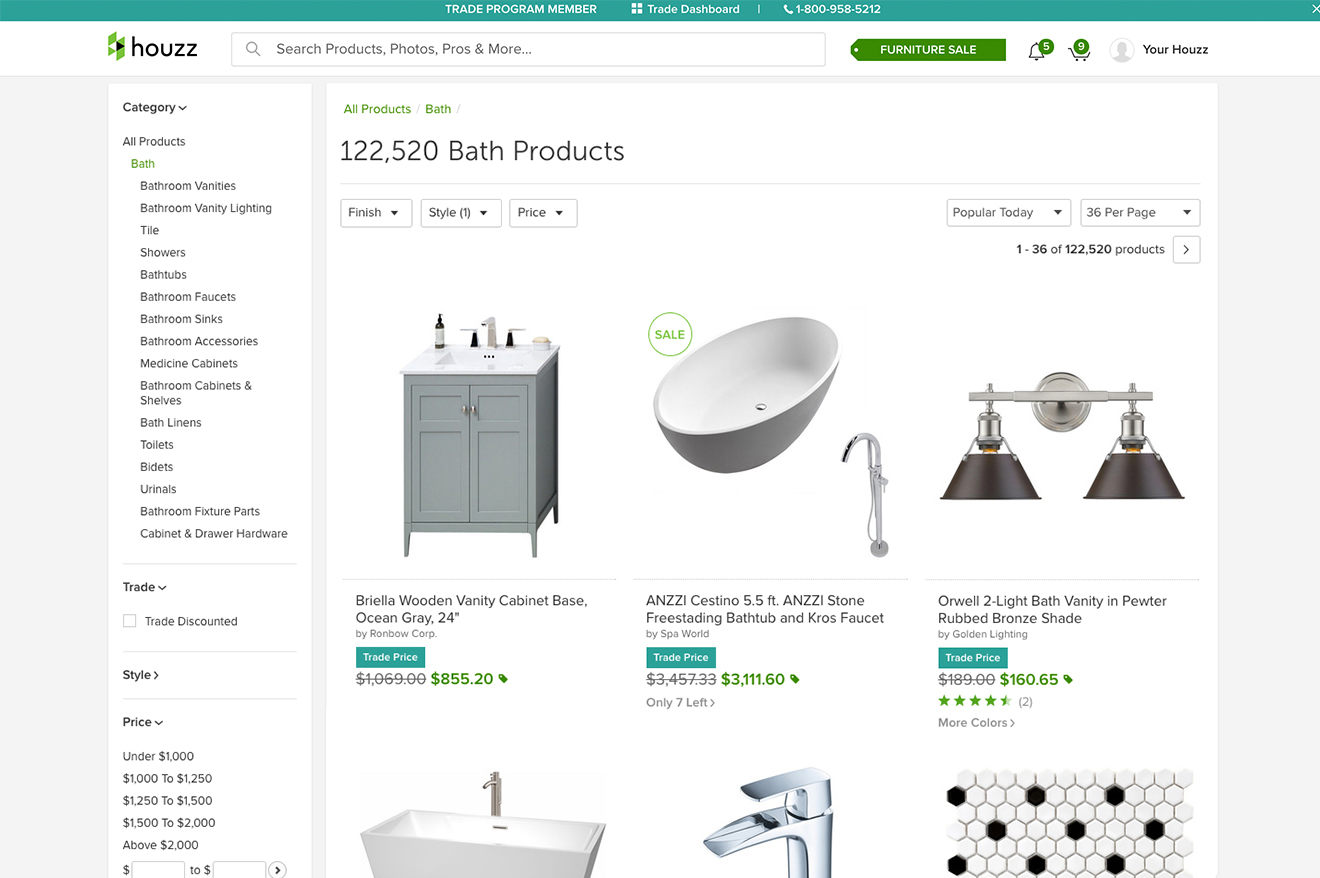This is a detailed screenshot of an e-commerce website named "Houzze" offering a variety of products for sale. The top of the page features a green navigation bar with three central links labeled "Trade Program Member," "Trade Dashboard," and a contact number formatted as a 1-800 number. Directly below, a white bar spans across the page displaying the website's name "Houzze" on the left in clear text, H-O-U-Z-Z-E, and a central search bar for efficient product queries.

To the right of the search bar, a prominent green tag indicates a "Furniture Sale," followed by a notification icon displaying five notifications in green, and a shopping cart icon showing nine items currently in the cart. Near these icons, a user profile button labeled "Your House" invites users to access their personal accounts.

On the left side of the page, a vertical white sidebar contains drop-down menus for filtering products by "Category," "Trade," and "Price." The main product area on the right side is organized with additional drop-down menus at the top for "Finish Style," "Price," "Popularity," and an option to display "36 per page." This structured layout facilitates user navigation, enabling efficient browsing and shopping experiences.